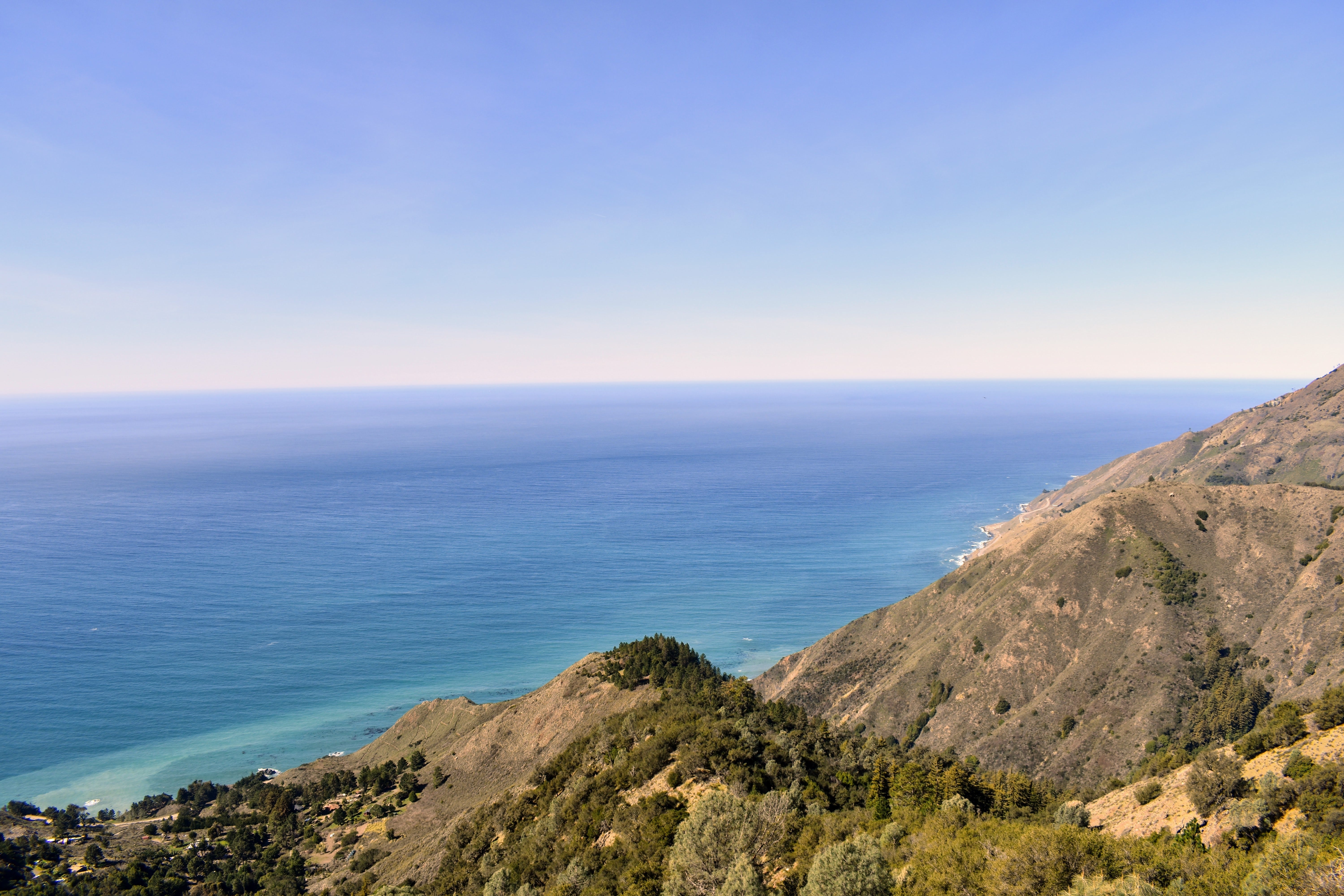This aerial photograph, likely taken from a drone or aircraft, captures a striking coastal landscape. Dominating the bottom right is a rugged mountainside covered with dense, green vegetation interspersed with patches of gray rock. To the left, the land flattens into a verdant area with a hint of a path or road amidst the trees. The coastline lacks a sandy beach, with rocky embankments plunging directly into the deep blue ocean, which transitions to a lighter blue closer to the shore. Offshore waters exhibit light wave action, suggesting deeper waters close to land. The image extends upwards to feature a vast expanse of the sky, showcasing a gradient that shifts from a deep blue at the top to a bright white at the horizon where it meets the serene ocean. The horizon line is clearly visible, giving a sense of depth and tranquility to the scene.